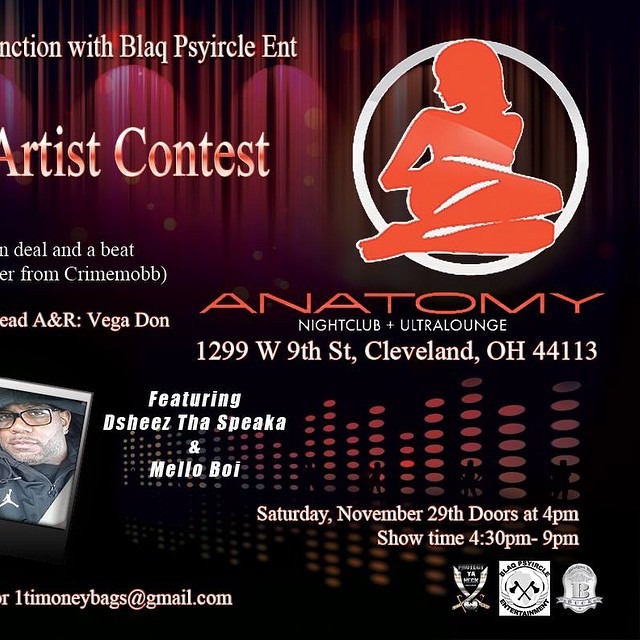The square image is an event advertisement for the Anatomy Nightclub and Ultra Lounge. It features a vibrant design with a red curtain adorned with various red and pink lights at the top. In the upper right corner, there is a reddish-orange illustration of a kneeling woman circled in white. Below this, the text "ANATOMY" appears in wide thin red font, followed by "NIGHTCLUB PLUS ULTRA LOUNGE" in smaller white capital letters. Positioned at the bottom left part of the image is a partial view of a black man in a black coat.

In the center of the image, the text announces the event details: "Saturday, November 29th, doors at 4 p.m., showtime 4:30 p.m. to 9 p.m." Additionally, it promotes an "Artist Contest" and features performers including DeShaz, The Speakah, and Mellow Boy.

At the bottom of the image are three logos, which are indistinct. The colors featured prominently in the poster are black, purple, pink, orange, white, and gray. The image appears to be an event poster, somewhat cut-off on the left side, making some text and details partially unreadable. An email address, something resembling "itmoneybags@gmail.com," is also mentioned, though it is difficult to read clearly.